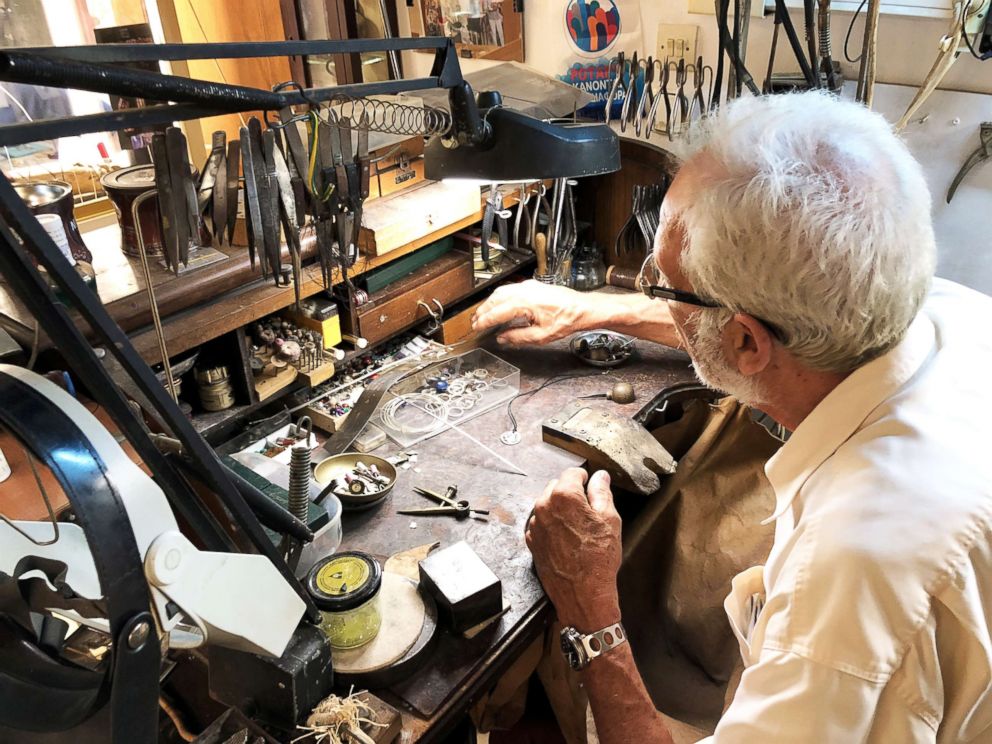The image depicts an older man, immersed in his work, seated at a cluttered wooden workbench that features numerous small drawers and an assortment of tools. He has short white-gray hair, wears glasses, and is dressed in a light yellow, almost off-white short-sleeved button-down shirt, with a silver wristwatch on his left wrist. The setting appears to be a garage, shed, or a dedicated workspace, characterized by the presence of various work materials including screws, nuts, bolts, and bowls. A black-colored lamp with a retractable fixture hangs above him, illuminating his work area. His left hand rests on the bench while his right hand reaches towards a drawer. The backdrop includes several hanging tools such as pliers and perhaps horseshoe-shaped items, while a large hammer can be seen hanging centrally. Attention to detail reveals other items like a glass cup containing yellow liquid and a light switch next to him. The colors in the image predominantly feature shades of black, gray, blue, yellow, and orange, adding to the intricate yet organized chaos of a busy workstation. The lighting in the image is ample, ensuring a clear and bright view of the scene.